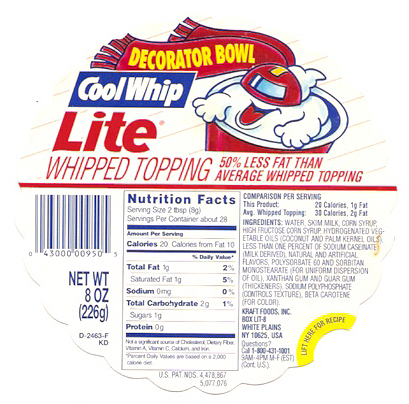This image showcases the top of a circular food container with scalloped edges. The container's design is vivid and informative. At the very top, the phrase "Decorator Bowl" is prominently displayed in yellow text, set against a red background that forms the scarf of a whimsical cloud cartoon character, which is positioned inside a red cup. Below this title, "Cool Whip" is prominently featured in white font on a blue background, with the word "Light" in striking red font adjacent to it. 

This indicates the product is "Cool Whip Light Whipped Topping," which boasts "50% less fat than average whipped topping," a detail that is printed to the right of the description. A barcode is located on the left side of the container's top, beneath which a red line delineates the product information section from the nutritional details. A box containing nutritional facts is situated to the right of the barcode, and a comprehensive list of ingredients can be found in the lower right corner. This detailed labeling provides consumers with all the essential information at a glance.